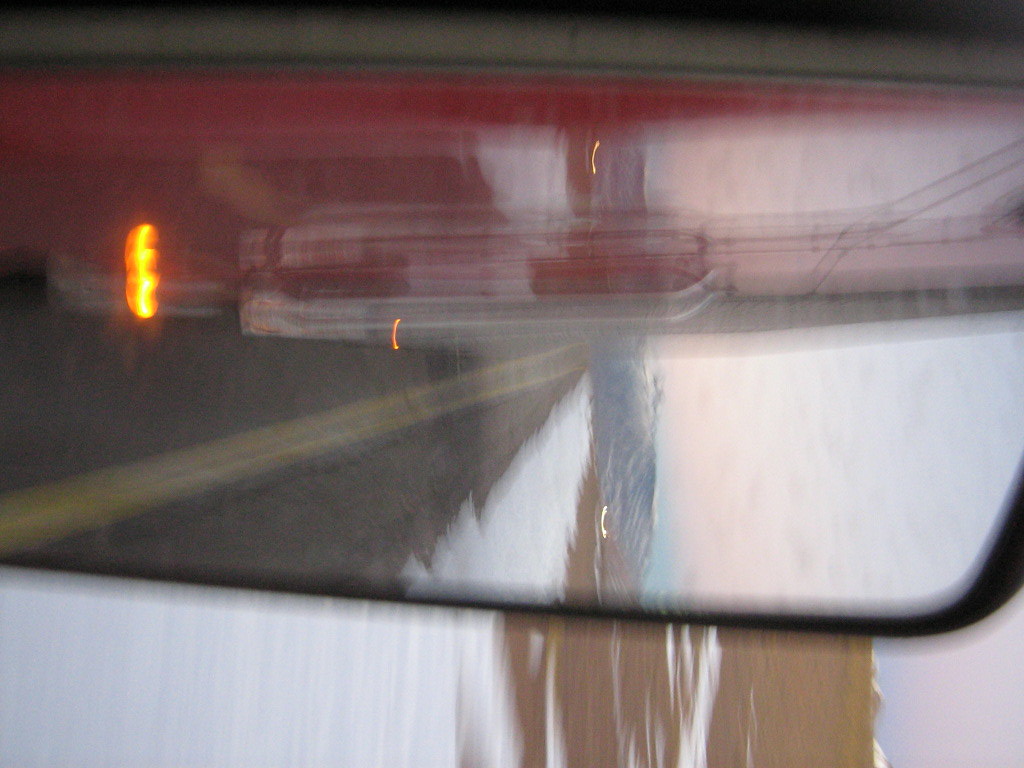In this color photograph, taken from an external side-view mirror of a red truck, the scene captured is a wintry landscape. The mirror, although partially cropped with its left side cut off, prominently displays a vibrant yellow light and an orange glow from an indiscernible source. The reflection reveals a light blue sky above a black mountain range. A black road containing a visible yellow line runs through the mirrored view, bordered by snow-covered ground and patches of frozen water. Behind the mirror, part of the truck’s red and silver body is evident, contributing to a blurry, chaotic visual composition. The upper right section outside the mirror frame is dusted with snow, accentuating the cold and frosty ambiance of the location.